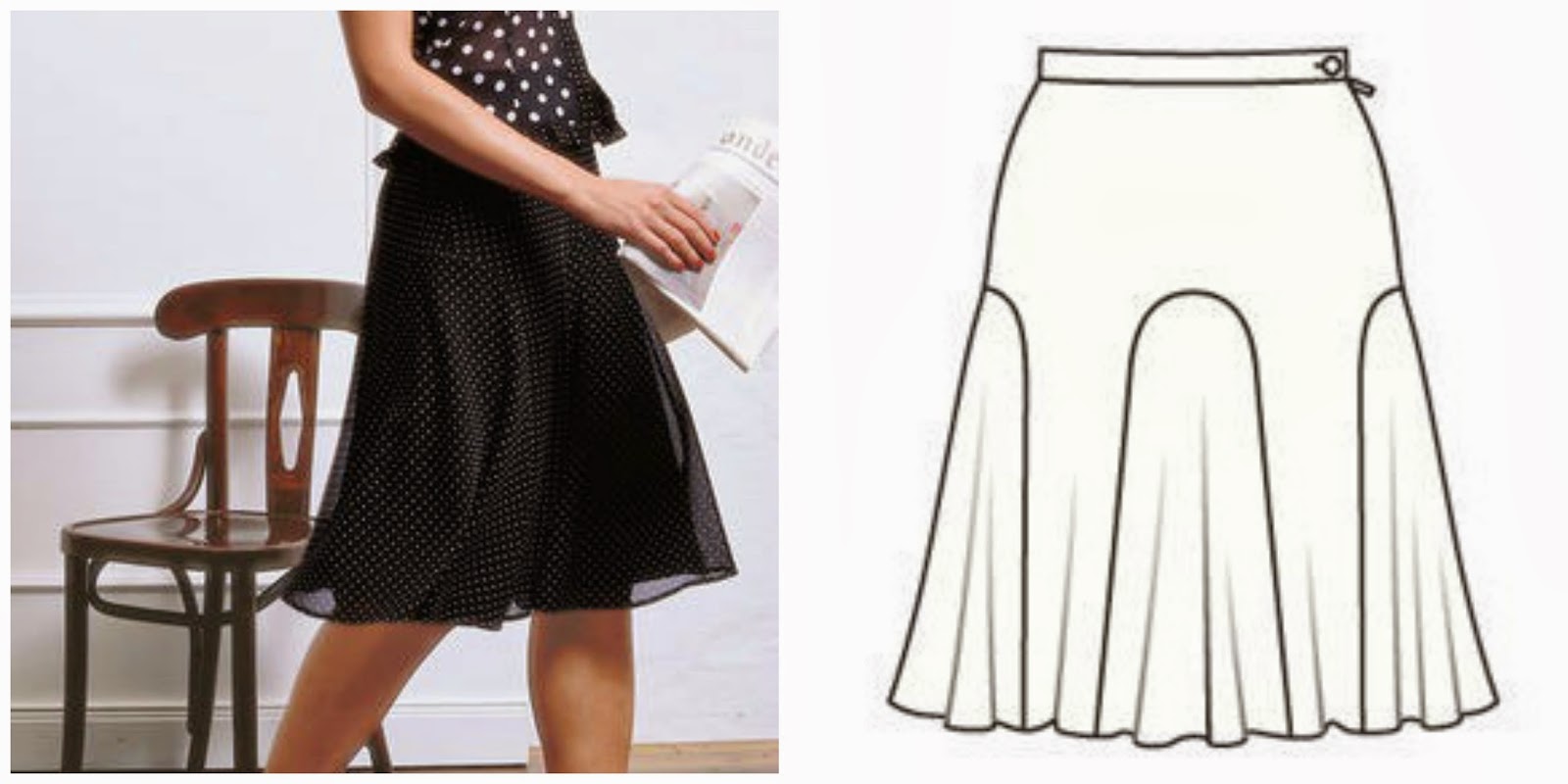The image is divided into two squares. The left square features a partial, real-life photograph of a Caucasian woman. She is shown from the top of her arm to her shins, wearing a black top with white polka dots and a full skirt that extends to just above her knees. The polka dots on her top are larger than those on her skirt. She is holding a newspaper in her right hand while walking. A white wall and a wooden chair can be seen in the background.

The right square presents a detailed black and white diagram of the woman's skirt, laid out on a white background. The diagram showcases the skirt's design, including elements like floral parts and archways at the bottom. The juxtaposition of these two images suggests that this might be a website or platform dedicated to showcasing patterns and designs for creating skirts.